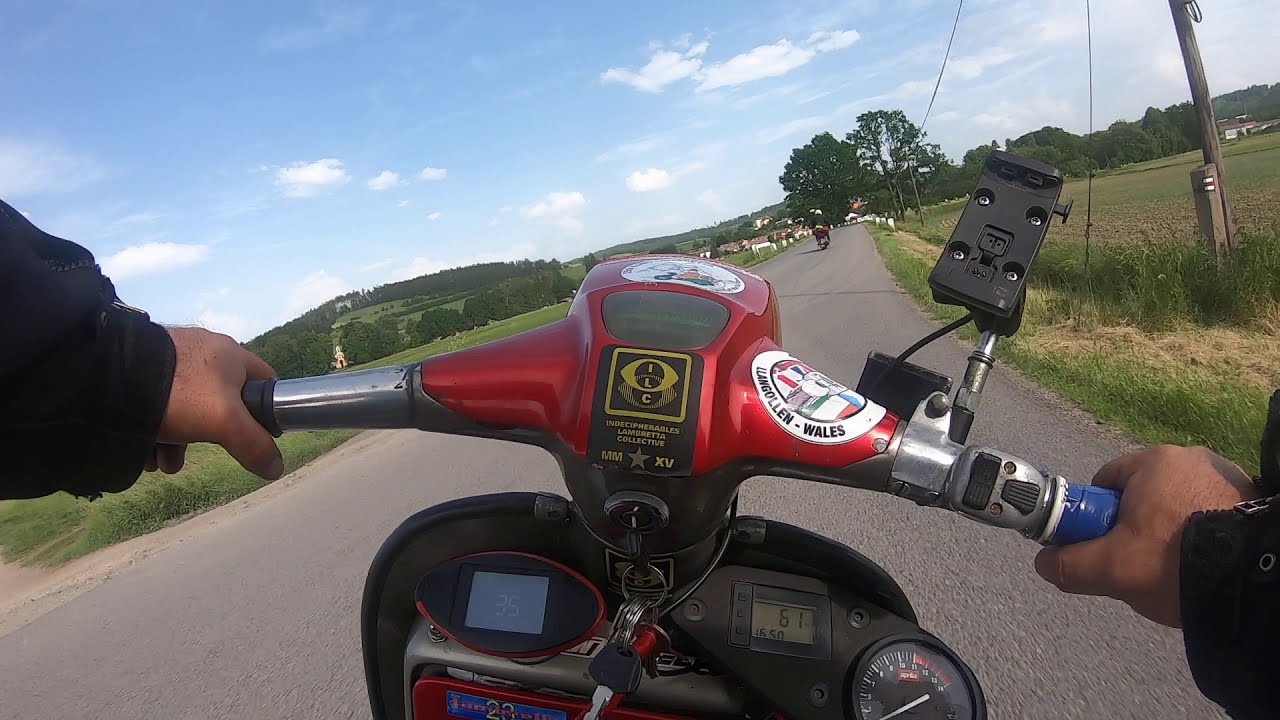In the photograph, a young man rides a red and silver scooter down an asphalt road in a rural area, with lush green trees and prairie land flanking both sides. He grips the handlebars firmly, visible alongside the scooter's odometer that displays numbers and a sticker bearing the word "Wales," suggesting a possible connection to the location. Ahead of him, another scooter and distant cars can be seen, hinting at fellow road users in this serene daytime setting. The expansive blue sky above is dotted with various types of white clouds, adding to the tranquil atmosphere. To the right, there is a field designated for crops, reinforcing the pastoral landscape, while tall grass grows along the road's edge. The man's attire is a black or gray jacket, and the scene captures the essence of a leisurely scooter ride through peaceful countryside terrain.